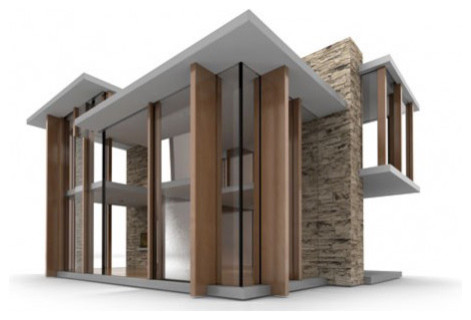This is a detailed 3D architectural rendering of a modern house, characterized by a sleek, angular design and an innovative use of materials. The structure prominently features large, single-pane floor-to-ceiling windows that dominate the frontage, providing a seamless connection between indoor and outdoor spaces. These massive glass panels are supported by perpendicular wooden dividers, which, in turn, uphold a flat, thick, off-white concrete roof. The facade combines elements of stone and concrete, with a substantial cobblestone wall serving as the central backbone of the design. This central wall extends vertically through both stories of the house, framing the structure and creating a strong visual anchor. The upper floor features an angular jut out, which is also glazed with heavy-duty looking glass and concrete, adding to the sense of modernity and robustness. The building’s palette includes tan, light orange, and off-white tones, complemented by the natural hues of the stone and wood. The roofline is flat with multiple tiers, and a potential balcony or covered patio can be seen on the less visible side, enhancing the functional outdoor living space. The design suggests a residence, albeit one with a very modern and narrow two-story layout, possibly even resembling a high-end office structure in its form and material usage.